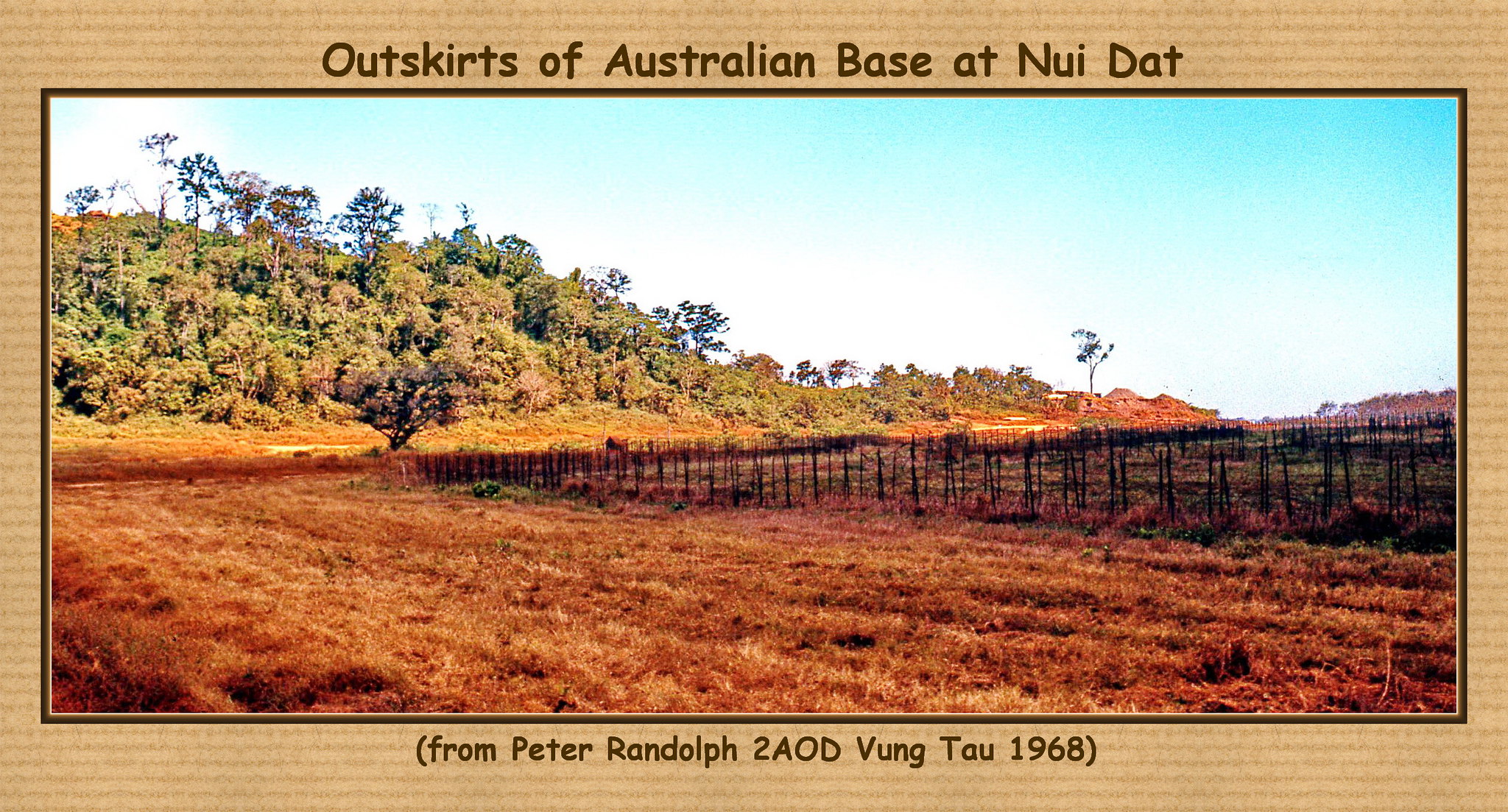This detailed postcard from 1968 features a color photograph capturing the "Outskirts of Australian Base at Nui Dat" in Vietnam, as indicated by the open black text at the top center. The landscape, bathed in daylight under a beautifully clear, aqua blue sky with white clouds, showcases the rural serenity of the time. The scene unfolds a rust-red soil field that might be part of a farm or plantation, with possible rows of crops outlined by fencing stretching across the image. On the mid-left, a small tree adds depth and frames the pastoral setting, with bushy green and brown vegetation sloping down from a hillside. In the background, there are clusters of trees: a prominent group towards the left and others distant on the top right. The postcard provides a sentimental touch through the text at the bottom, "From Peter Randolph to AOD Vung Tau, 1968" in parentheses, offering a glimpse into a personal connection during the Vietnam War. Surrounding the photograph, the postcard has a soft, light cocoa-brown border, adding a nostalgic texture to this historical snapshot.